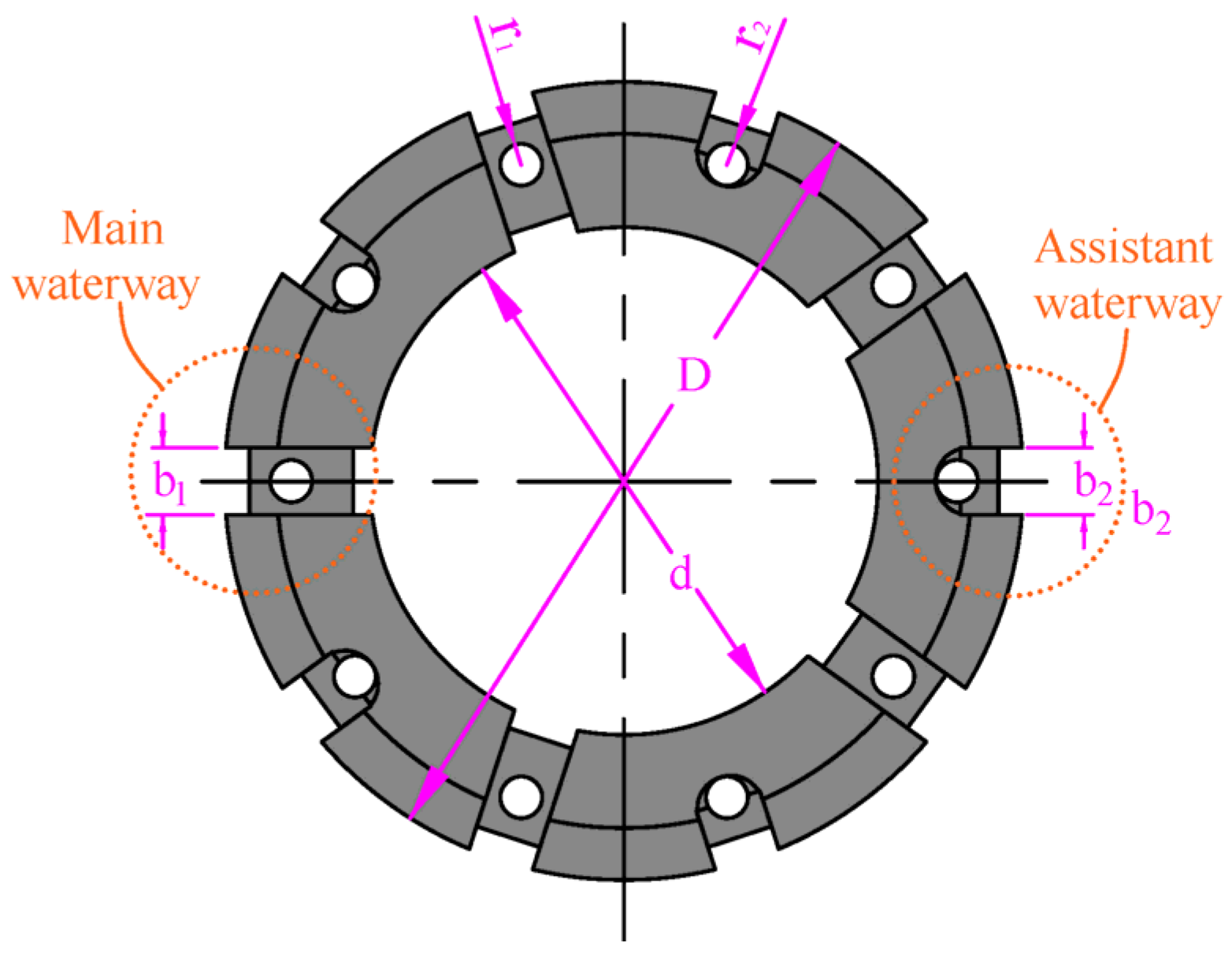The image is a detailed color illustration of a gear-shaped object on a white background, resembling a scientific diagram. The central element is a gray circular gear with eight white holes arranged in a ring around the center. There are numerous purple arrows labeled with uppercase and lowercase letters, including D, pointing in various directions across the circle. The gear is divided into quadrants, with intersecting lines running from top to bottom and left to right. 

On the left side of the diagram, there is an orange-labeled section marked as "Main Waterway," highlighted by an orange circle and accompanied by an arrow pointing towards this part of the gear. Similarly, the right side features a section labeled "Assistant Waterway" in orange, also circled and connected by an arrow. The illustration blends clear typography with color coding to indicate different parts and functions, creating a comprehensive and detailed visual representation of a complex waterway or mechanical system.